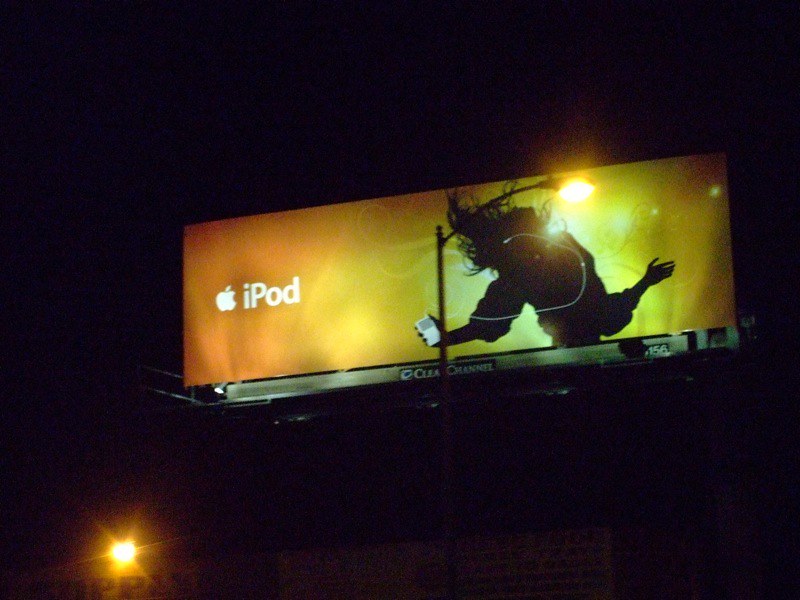The photograph captures a nighttime street scene with a prominent billboard advertising the Apple iPod. The large rectangular billboard, illuminated to stand out against the dark night sky, features a striking design with an orange and yellow gradient background. On the left side of the billboard is the iconic white Apple logo followed by the word "iPod." Dominating the right side is a black silhouette of a woman with long hair, who is dancing with her head tilted back, clearly enjoying the music. Her white iPod and the connected white earbud wire are vividly highlighted against her dark figure. The billboard is partially obstructed by a tall, standard streetlight positioned directly in front of it, casting a glow that hinders part of the image. Additionally, a bright amber-colored light at the bottom of the scene illuminates an obscure sign, adding to the urban nighttime ambiance.